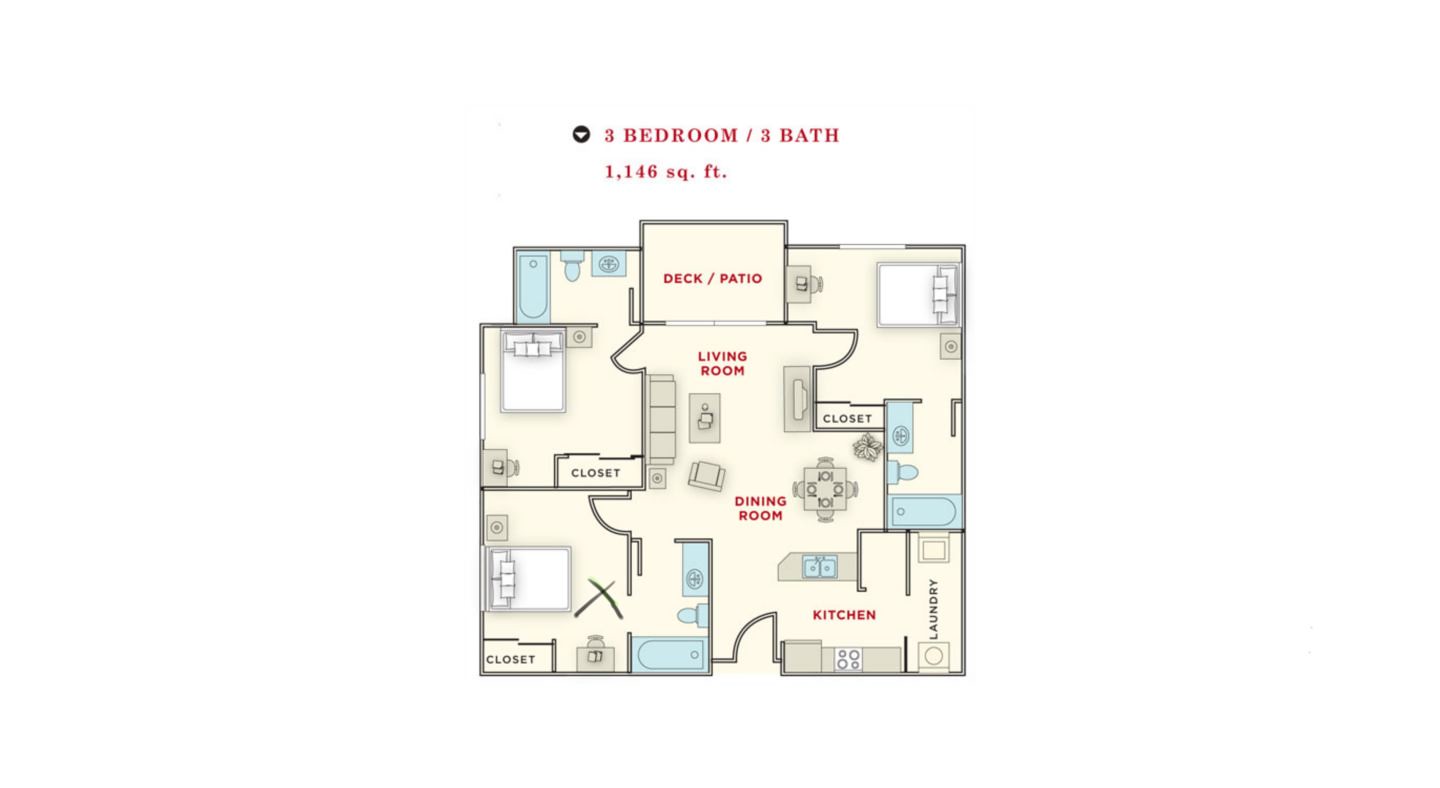**Detailed Caption:**

The image illustrates a digitally-created floor plan of a home. Dominating the visual is a white background, against which the floor plan is presented in a light yellow-beige hue. At the top of the image, there is a prominent black circle featuring a white downward-pointing triangle. To the right of this symbol, in the center of the image, bold red capital letters spell out "3 BEDROOM / 3 BATH." Directly below this, in smaller red lettering, it indicates "1,146 SQUARE FEET."

The layout includes comprehensive labels in various colors. Living spaces and key areas are highlighted in red capital letters, with furniture rendered in a khaki shade and outlined for clarity. Centrally, "LIVING ROOM" is clearly marked, and above it, the "DECK / PATIO" is labeled at the top middle section of the plan. 

Bathroom amenities, such as toilets, sinks, and baths, are illustrated in blue, with a total of three visible in the blueprint. The kitchen is situated at the bottom right and labeled prominently in red capital letters. Adjacent to the kitchen, in the lower right-hand corner, is the laundry room, uniquely labeled in black letters.

The home includes three bedrooms, each furnished with a closet: one bedroom is located at the top right, another at the bottom left, and the third centrally on the left side of the plan. Entrances and additional storage spaces include three clearly marked closets. The front door is positioned at the bottom center, providing entry to the home.

Room divisions and the entire structure are defined by walls in a dark grayish-green color, giving a distinct separation to each area of the layout. This floor plan meticulously details the home's arrangement, making it easy to visualize the spatial organization.